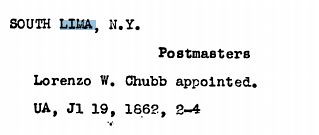The image features an old telegraph with a white, empty background. The text on the telegraph, which appears to be typed with an old-school typewriter, reads: "South Lima, New York. Postmasters. Lorenzo W. Chubb, appointed. U.A. J.I. 19, 1862, 2-4." The text is predominantly in black except for one word highlighted in blue. The date likely indicates February 4th, 1862, suggesting the appointment of Lorenzo W. Chubb on that day.